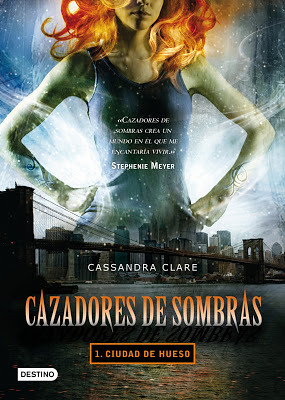This poster, likely for a movie or a book adaptation, features a vibrant and dynamic image of a woman with fiery red, wavy hair standing confidently with her hands on her hips, dressed in a black sleeveless tank top. She appears almost superhero-like, positioned prominently above a cityscape that closely resembles New York with its iconic skyline and large bridge extending over a waterway. The background adds a colorful and intense atmosphere, akin to a bat signal.

Central to the poster are various texts. Across the top, there's white text in a foreign language and the name "Stephenie Meyer". Below it, "Cassandra Clare" is prominently displayed. The title "Cazadoras de Sombras" is rendered in a striking gradient font that transitions from orange at the top to nearly white at the bottom. Beneath this, within a black box outlined in orange, is the text "1 CIUDAD DE HUESO".

In the bottom left corner, a white arrow-like mark points right next to the black text "Destino" on a white background, suggesting a navigational element or a projected detail.